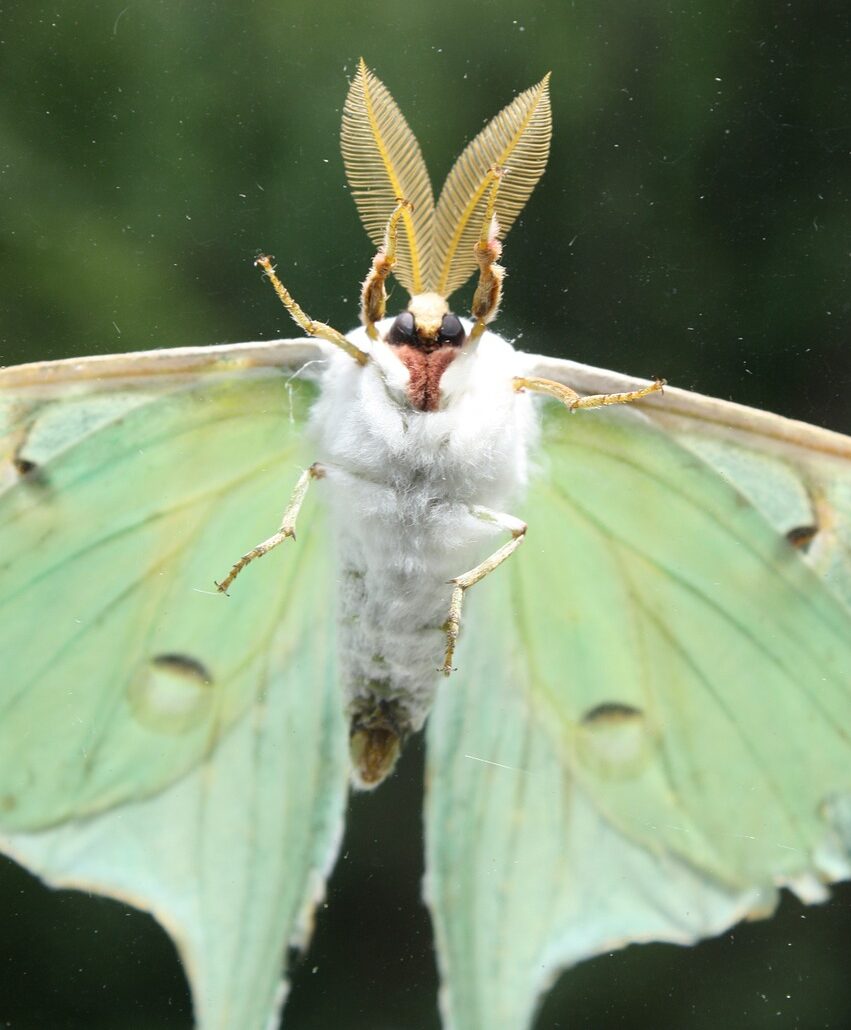The image is a close-up of a captivating moth, centrally positioned to highlight its detailed features. The moth boasts a fluffy, white furry body with its legs splayed out as if in mid-flight. It has mesmerizing black eyes that stare directly at the viewer and uniquely leaf-shaped yellow antennas that rise from its head. The wings are a tranquil seafoam green with light jagged edges, hinting at their delicate structure. The background is artistically blurred, giving just a shade of green, which suggests a natural, leafy environment. This exquisite insect combines elements of both elegance and intrigue, standing out with its distinctive appearance in a dark green backdrop.